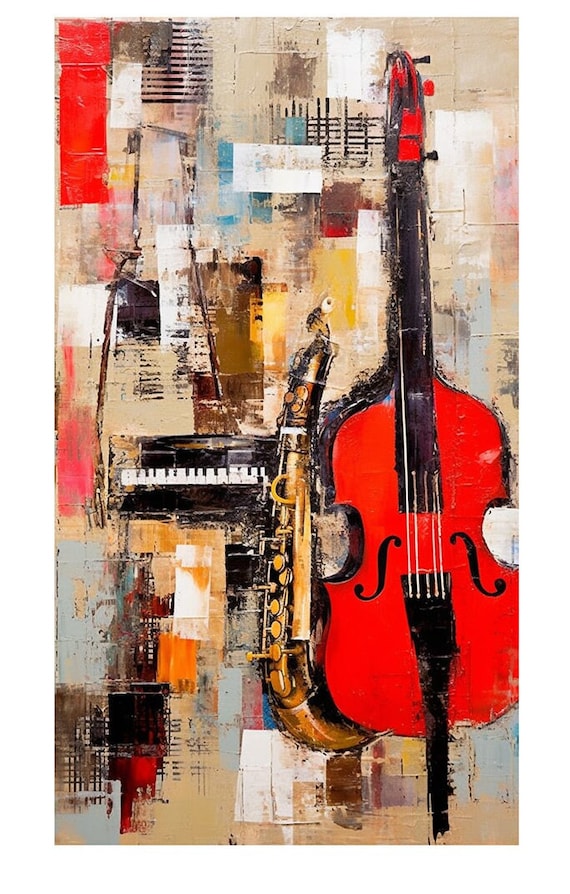This vibrant and tall abstract painting melds several musical instruments into an intricate, quilt-like composition of colors and patterns. Dominating the right-hand side is a bright red violin or cello, stretching from the top to the bottom of the image. Adjacent to it, a brass saxophone or clarinet takes center stage, flanked on the left by a small section of a piano keyboard with its distinctive black and white keys. The background features a hodgepodge of colors—whites, oranges, pale hues, reds, and blues—arranged in checkered and grid patterns. These colorful squares and artistic flourishes form an abstract mosaic that emphasizes the musical theme. The entire composition is devoid of any writing, people, or animals, focusing solely on the blend of musical elements and modern art.